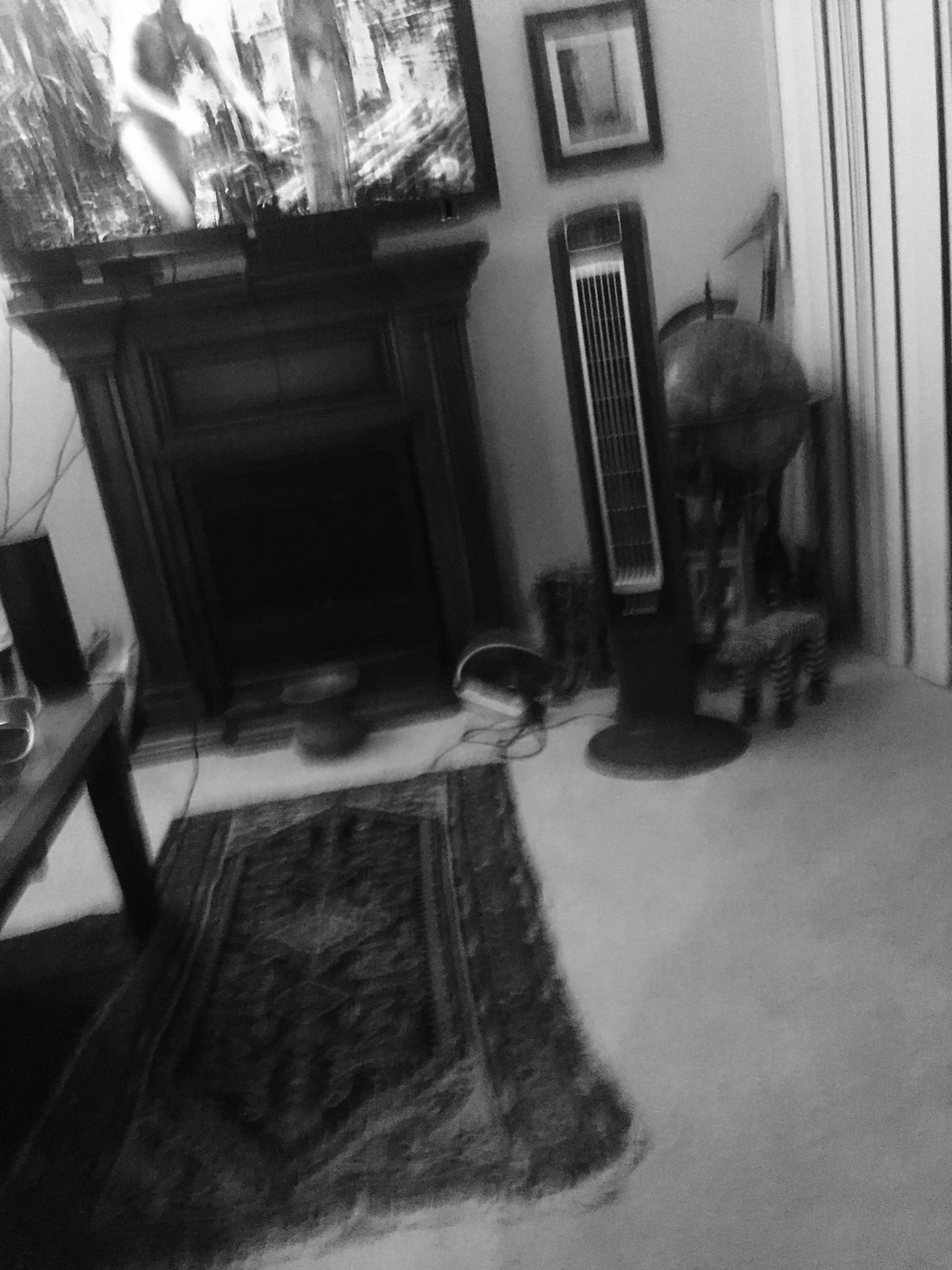This detailed black-and-white photograph captures an eclectic living room interior. The focal point is a very narrow, dark wooden fireplace that appears non-operational, adorned with a small mantle. Above the mantle, there's a screen displaying an image of a person riding a bike, possibly a TV, alongside an 8x10 hanging picture. In front of the fireplace, a jar or pot rests on the floor, along with a small, ornate oriental-style rug featuring fringed edges and various intricate patterns.

To the right of the fireplace stands a tower-like fan or electric heater, with a large standing globe and a stylized carving of a cat, potentially a zebra statue, positioned behind it. Additional wires snake across the floor and wall from this corner. To the left, partially visible, is a portion of a table or desk scattered with objects, further cluttered with wires that may connect to extra speakers or a surround sound system. The room's flooring is a simple beige carpet, providing a neutral backdrop to the otherwise richly detailed and somewhat cluttered interior.